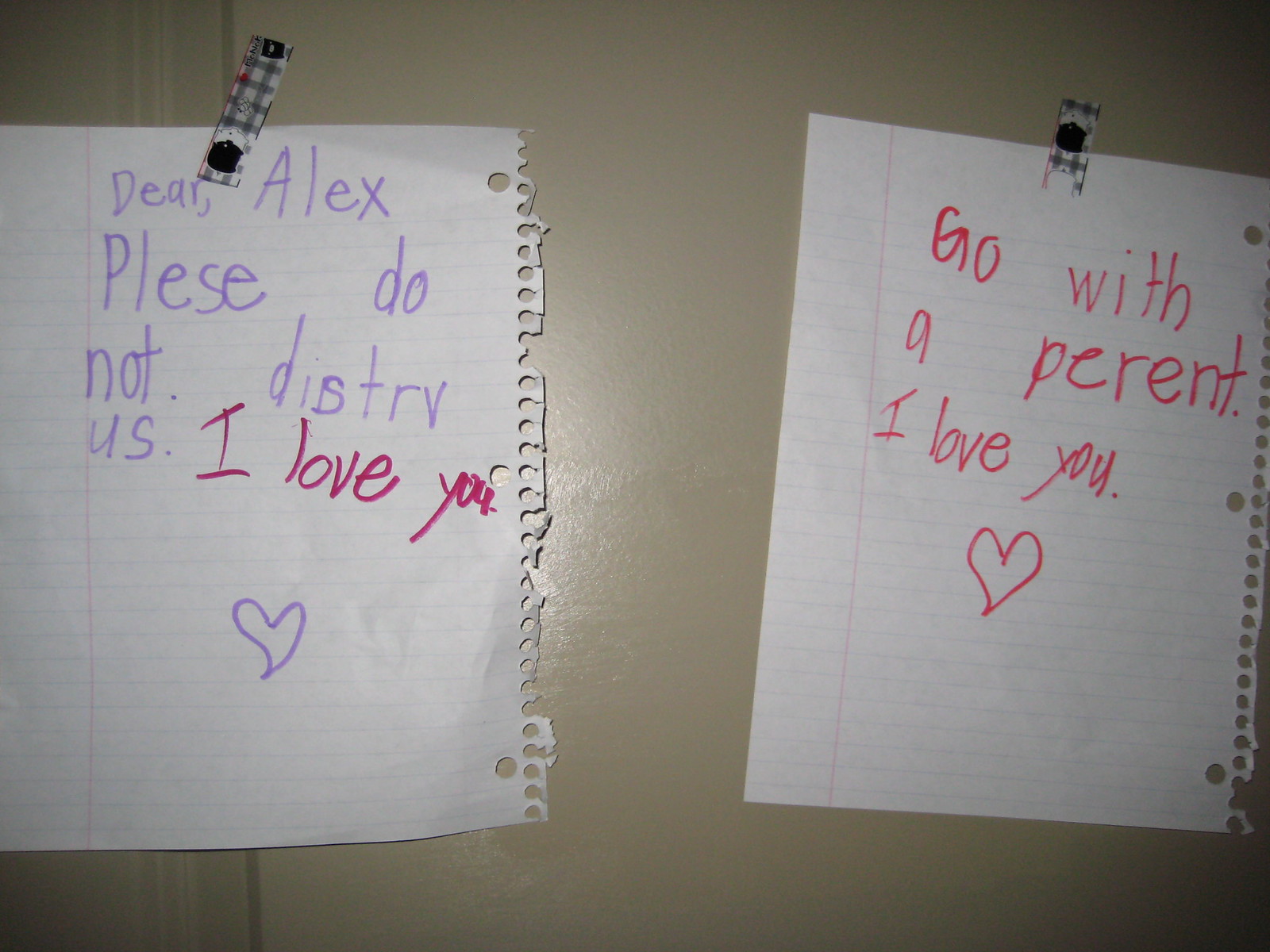The image depicts two pieces of white notebook paper, complete with the characteristic blue lines and the torn edges from where they were ripped out of a spiral notebook, taped to a tan-colored wall. 

On the left piece of paper, written in purple ink, is a heartfelt message: "Dear Alex, please do not destroy us. I love you," accompanied by a small heart at the bottom. The word "please" is misspelled as "P-L-E-S-E," indicative of the writing likely coming from a young child, possibly a third grader. 

The right piece of paper has a message written primarily in red ink, reading "Go with a parent. I love you," with another hand-drawn heart beneath. The handwritten messages, though somewhat difficult to decipher due to the childlike script and occasional misspellings, convey a sincere and touching sentiment from the young author.